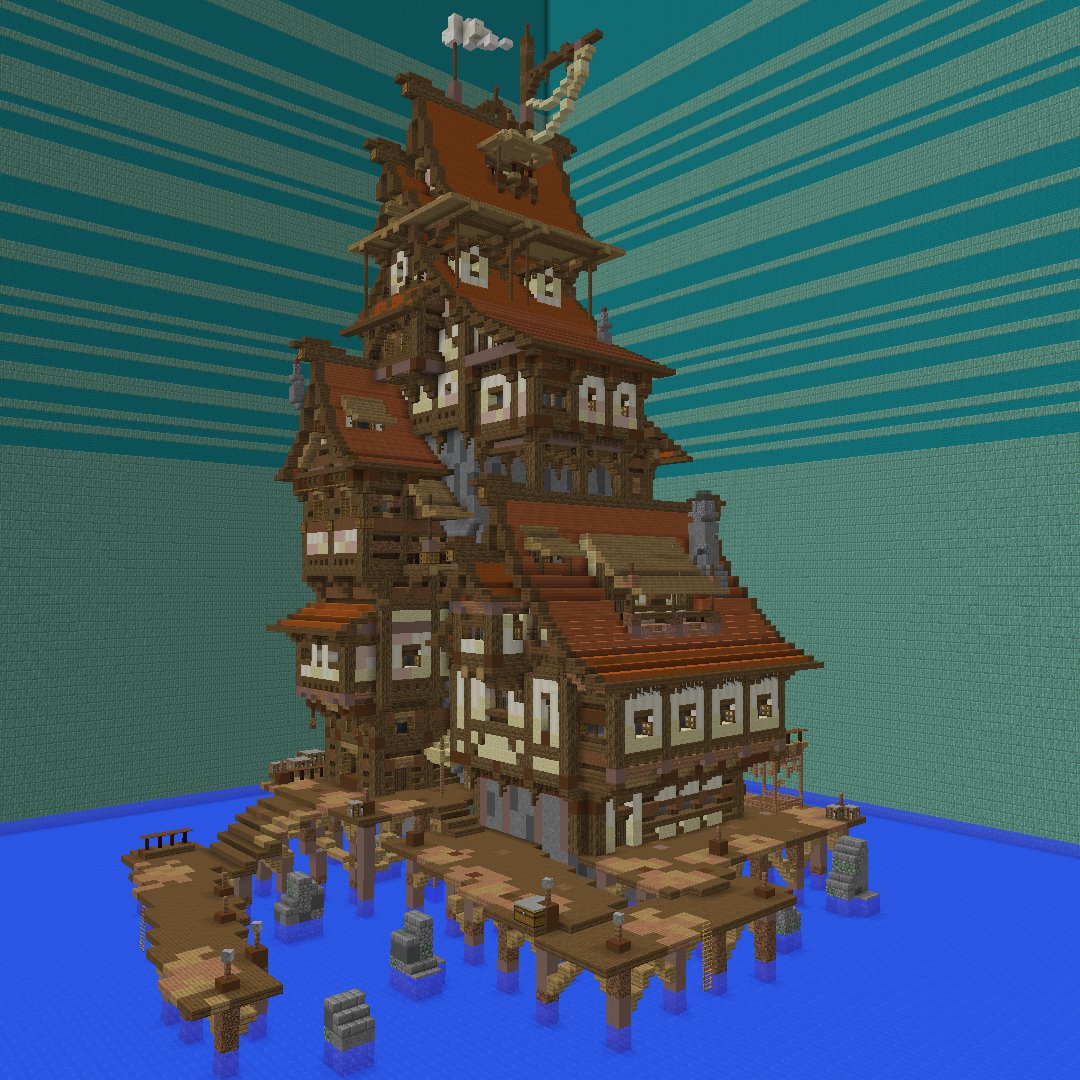This outdoor image appears to be a highly detailed, computer-generated graphic reminiscent of a Minecraft design. It features a complex, multi-level house, appearing as if constructed from Legos, situated on pillars that are sunken into a shallow, bright blue expanse of water. The main structure consists of three distinct sections, seemingly merged into a single tower with a flag at its peak. The first structure is a gray, three-story building with red gabled roofs. Attached to it is a taller tower composed of several house-like attachments, each with rich mocha brown gabled roofs, bordered in darker brown. The interconnected buildings share a platform that extends to a wooden deck with brown steps leading down to the water. The background features walls at a 90-degree angle to each other, adorned with teal horizontal streaks, set against a pixelated, green backdrop.